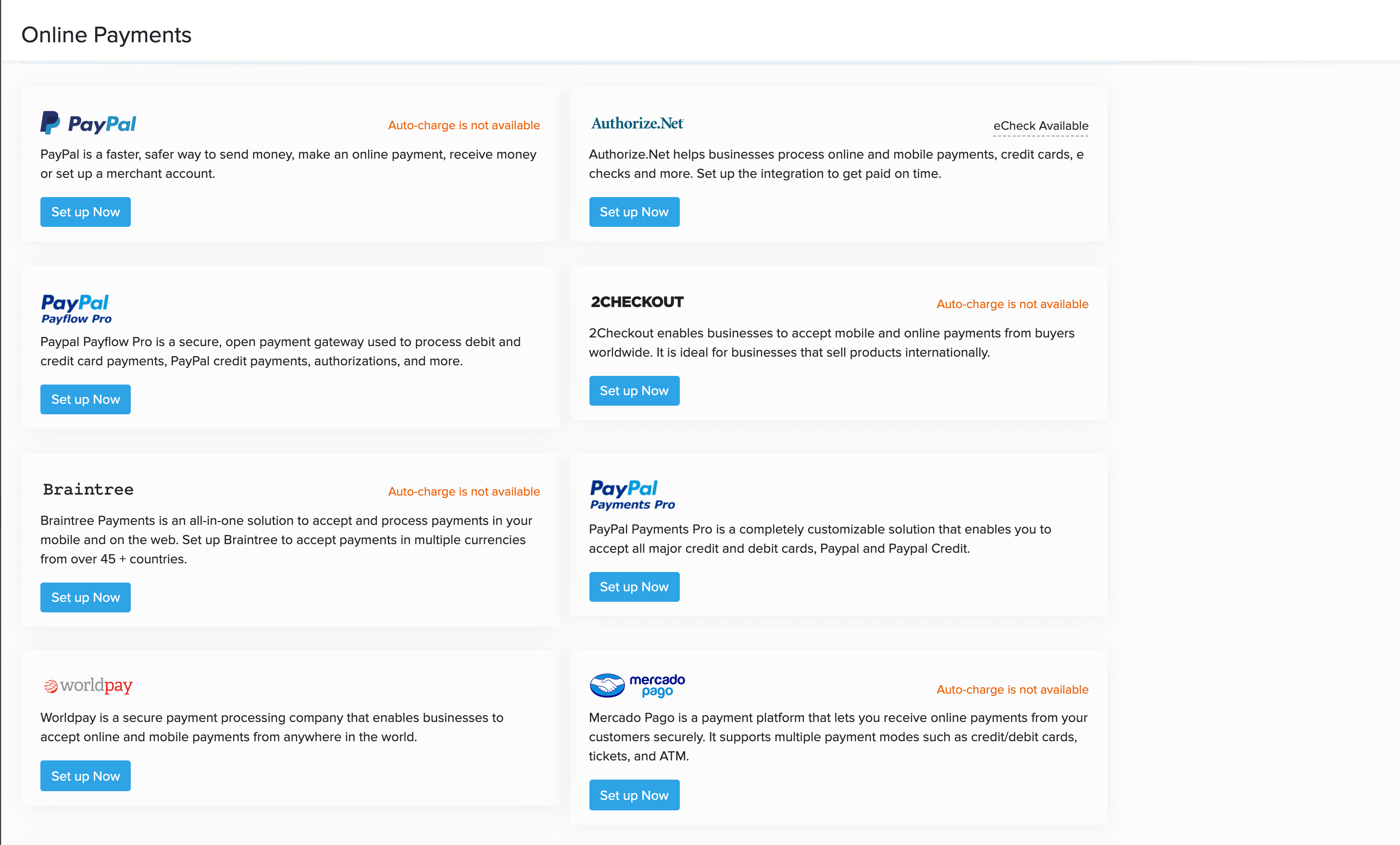This is a detailed screenshot from the PayPal website, highlighting various online payment options. At the very top of the page, the title "Online Payments" is displayed in black letters. Below the title, there are eight distinct categories, each encapsulated in a white rectangular box, arranged in two columns, four on the left and four on the right.

### Left Column:
1. **PayPal**: This option includes orange text stating "auto charge is not available." Below a brief description of PayPal, there is a blue rectangular "Set Up Now" button in white text.
2. **PayPal PayFlow Pro**: Like the PayPal option, it also features a "Set Up Now" button in blue with white text.
3. **Braintree**: This category specifies in orange text that "auto charge is not available" and also includes a "Set Up Now" button.
4. **World Pay**: The word "World" appears in gray text, while "Pay" is in red text. This category too includes the "Set Up Now" button.

### Right Column:
1. **Authorize.net**: Featured in blue text, with "E-Check Available" indicated on the far right.
2. **2Checkout**: Displayed in black text with an orange notice to the right stating "auto charge is not available."
3. **PayPal Payments Pro**: This is another PayPal-related option included for setup.
4. **Mercado Pago**: Presented in blue text, it accompanies an orange note that "auto charge is not available." Additionally, it features a logo to the left, depicting two white hands shaking each other within a blue circle or oval.

Each category ends with its respective "Set Up Now" button, maintaining a uniformity throughout the page.